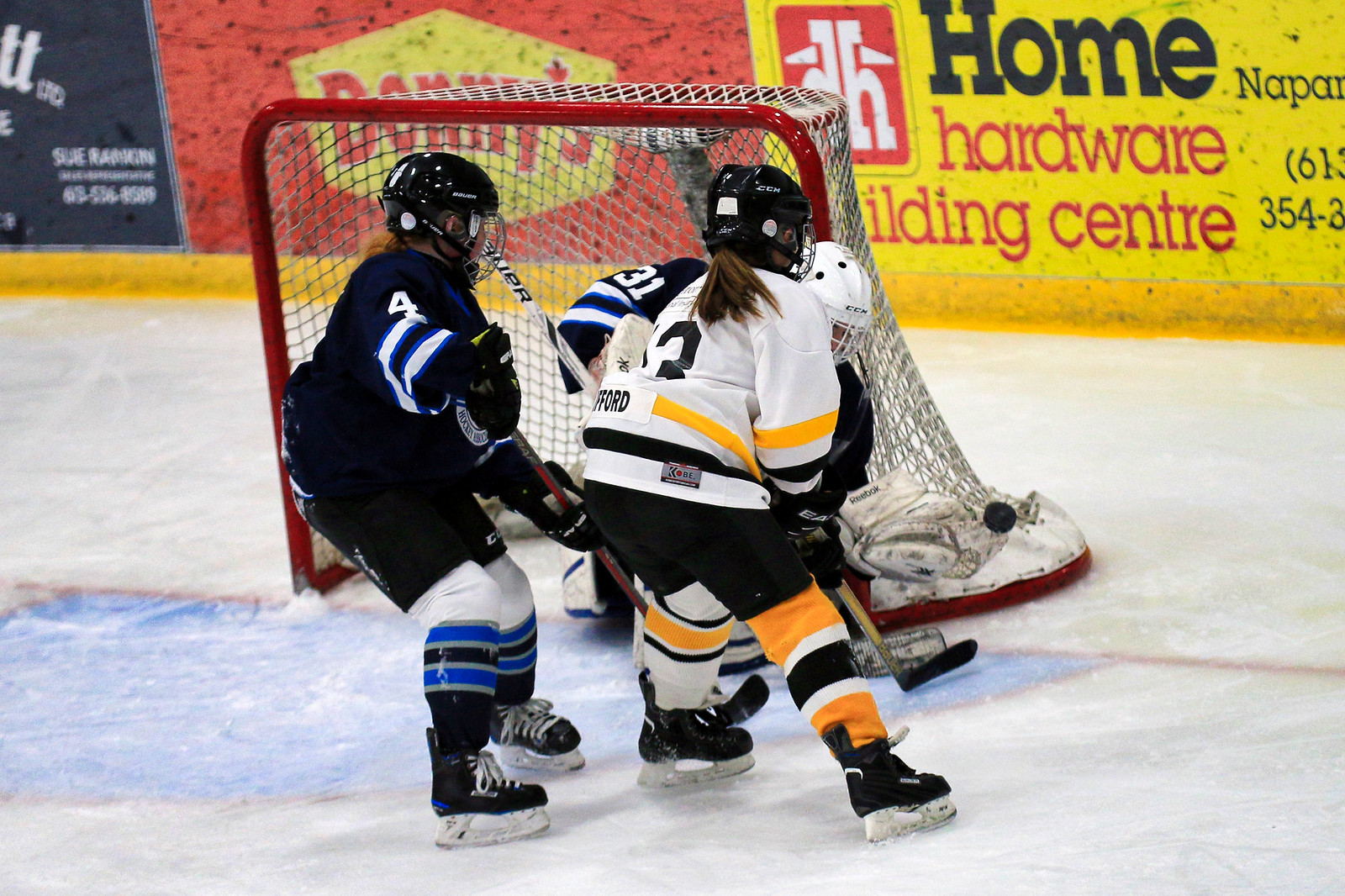The photograph captures an intense moment in an ice hockey game, featuring three players and the goal. The goalie, wearing a dark jersey with blue and white stripes and a white mask and helmet, is positioned in front of the white net framed in red metal, facing towards the camera. Her teammate, also in a dark jersey and helmet, assists from nearby. They are defending against an opponent trying to score, who is dressed in a mostly white uniform with black and gold accents. The puck is visibly flying off to the right as the goalie makes a defensive play.

In the background, several advertisements line the rink’s panels. Prominently displayed are signs for Denny's Restaurant in red and yellow, and Home Hardware Building Center in yellow with red and black text, including part of a phone number (354). Another partially visible sign mentions "Sue Rankin" along with a phone number cut off at the edge of the image.